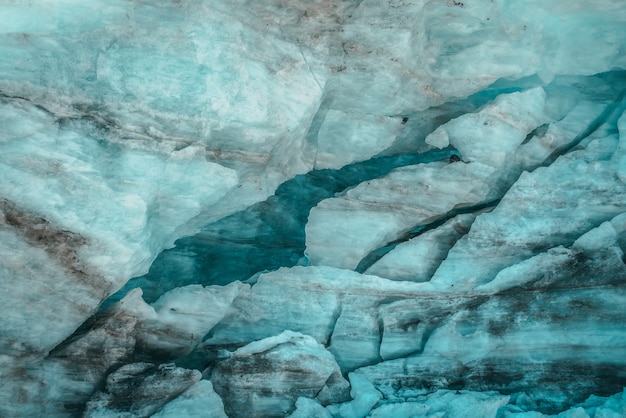This outdoor photograph captures a close-up view of a dirty and cracked glacier, presenting a detailed and textured landscape. The glacier's surface is predominantly a bluish-white, with substantial cracks running through it, the most notable being a deep, prominent fissure extending from the bottom left to the top right, which reveals a darker blue hue due to the depth and reduced light. The image suggests the presence of a central cavern filled with bright blue water, flowing through the glacier, with the surrounding ice showing significant dirt and sediment accumulation, particularly in the bottom corners. While the top part of the glacier retains some crystalline white areas, the bottom sections are muddied, with black grains and dirt mapping the glacier’s interaction with the underlying rocks and sediments. The photograph provides an intimate glimpse into the glacier's structure and the impacts of erosion and sedimentation.